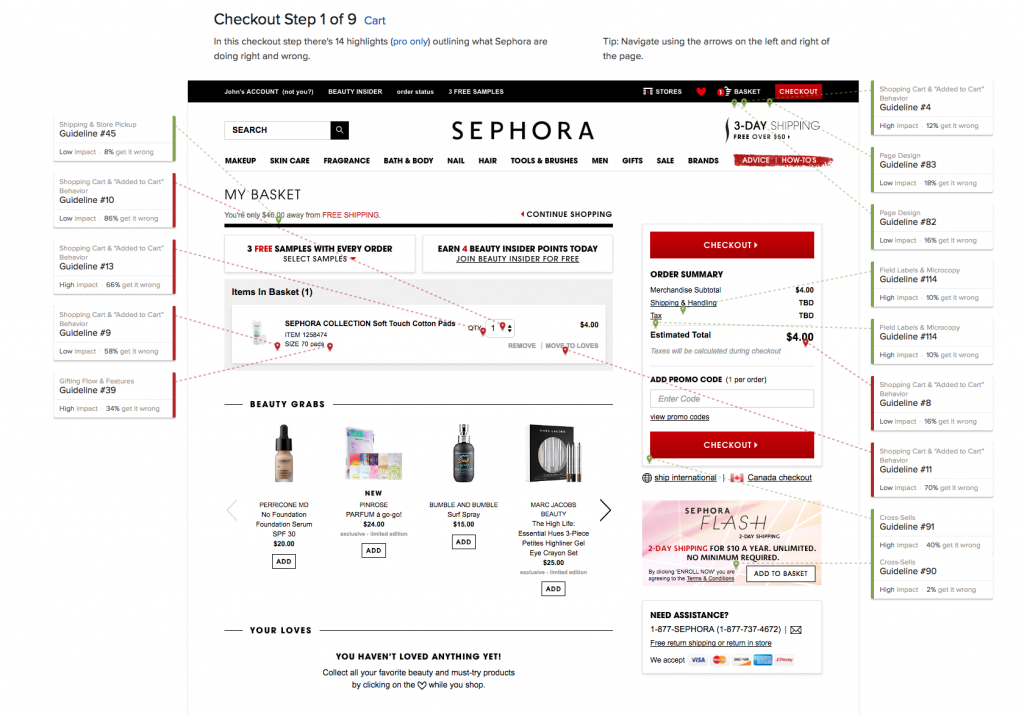**Detailed Annotated Screenshot of Sephora Website for Internal Analysis**

In this detailed screen grab of the Sephora website, designed for an internal analysis for designers or project teams, various elements of the checkout process are annotated and evaluated. The central focus of the image prominently displays Sephora's website, highlighting the user's shopping cart and order summary. The page features an array of products, making up approximately 80% of the graphic.

**Top Section: Checkout Process Overview**
- The top of the screen outlines the current step in the checkout process: **"Checkout Steps: 1 of 9 – Cart"**. 
- Instructions are provided on navigating the page using arrows on the left and right, marked as a tip.

**Annotations: Analyzing User Flow and Design Effectiveness**
- **14 highlighted areas** are marked on the page, pointing out specific design elements and user flow aspects.

**Green Annotation Box: Positive Highlight**
- **Guideline #44: Shipping and Store Pickup** 
  - *Impact:* Low 
  - *Statistics:* 8% get it wrong
  - A green box, indicating positive feedback, points to the message: **"You're only $46 away from free shipping."**
  - *Analysis:* This is praised for encouraging users to add more items to qualify for free shipping, effectively driving additional sales.

**Red Annotation Box: Negative Highlight**
- **Guideline #10: Shopping Cart and Added to Cart Behavior**
  - *Impact:* Low
  - *Statistics:* 86% get it wrong
  - A red box, indicating an area for improvement, points to the user's basket where the quantity is displayed as "1" with a selectable box.
  - *Analysis:* This suggests that Sephora's current implementation of adding items to the cart may not be user-friendly and is recognized as a common issue among similar sites.

**Additional Annotations**
- Several other green and red annotation boxes identify more areas where Sephora's website design either excels or requires enhancement. These are systematically labeled with corresponding guideline numbers and impact statistics.

This thorough analysis is crucial for refining user experience and optimizing the website's checkout process, ensuring both seamless navigation and heightened customer satisfaction.